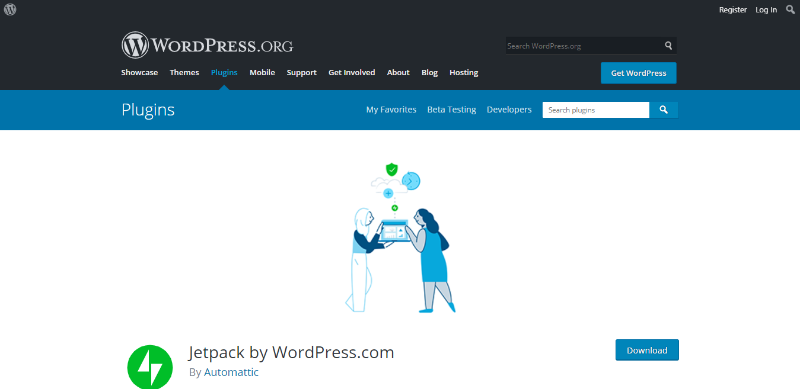This is a detailed screenshot of the WordPress.org website interface.

At the top of the screen, there is the WordPress logo, a bold black "W" inside a white circle. Adjacent to this logo is the search bar labeled "Search WordPress.org," allowing users to find specific content on the site. Following the search bar, there is a blue "Get WordPress" button with white text that enables users to download the platform.

The primary navigation menu is presented on a solid black background with white text for each menu item. However, the current page, "Plugins," is highlighted in bright blue. The navigation menu includes the following headings: 
- Showcase
- Themes
- Plugins (highlighted in blue, indicating the currently active page)
- Mobile
- Support
- Get Involved
- About
- Blog
- Hosting

Beneath this navigation menu is a dropdown section specifically for "Plugins." This section is set against a vivid blue background, lighter than navy, and contains white text. It is organized with the following headers:
- Plugins
- My Favorites
- Beta Testing
- Developers

In this dropdown section, there is a search box with grey text indicating "Search plugins" and a magnifying glass icon for initiating the search.

Additionally, the screenshot features an image of two women, each holding a laptop. One woman is dressed in pants while the other wears a dress. Their laptops emit illustrated lines and dots reminiscent of thought bubbles and pictures, symbolizing the exchange of ideas and content.

Beneath this illustration is a section for "Jetpack by WordPress.com," developed by Automattic. This section includes a green logo with white text and a blue "Download" button.